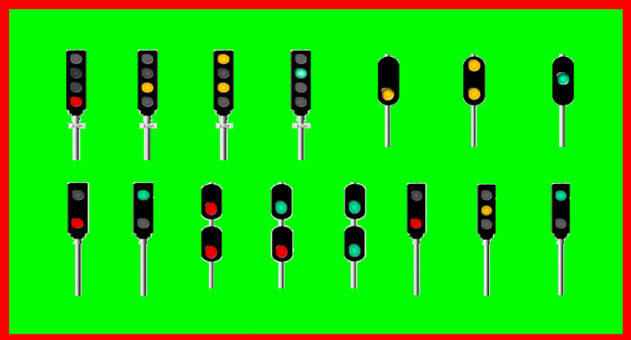The image, resembling digital art or an old computer graphic, features various types of traffic lights arranged in a horizontal rectangular format with a thin, bright red border and a neon green background. It contains two horizontal rows of traffic lights, with seven lights in each row, summing up to fourteen distinctly designed yet similar traffic lights. 

In the top row, the first four traffic lights are vertical black rectangles with four circular lights each, but feature different lit sections:
1. The bottom light is red.
2. The second-from-bottom light is yellow.
3. Two yellow lights are lit in the second and fourth positions.
4. The third position light is green.

Following these, the next three lights in the top row transition to a smaller rounded rectangular shape:
5. The bottom light is yellow.
6. Both the top and bottom lights are yellow.
7. The middle light is green.

In the bottom row, the shapes and configurations vary further:
1. Two identical vertical rectangles with two lights each; the bottom light is red.
2. The top light is green.
3. Two black ovals stacked vertically on the same pole, both displaying red lights.
4. Similar double-stacked ovals with the top light green and the bottom light red.
5. Another set of double-stacked ovals, both showing green lights.
6. A vertical rectangle with a red light on the bottom.
7. A rectangle featuring a yellow light in the middle position.
8. The final light is a rectangle with the top light green.

All traffic lights have circular lit areas, creating a visually striking and varied array of traffic signals in vivid, eye-catching colors against a stark neon backdrop.